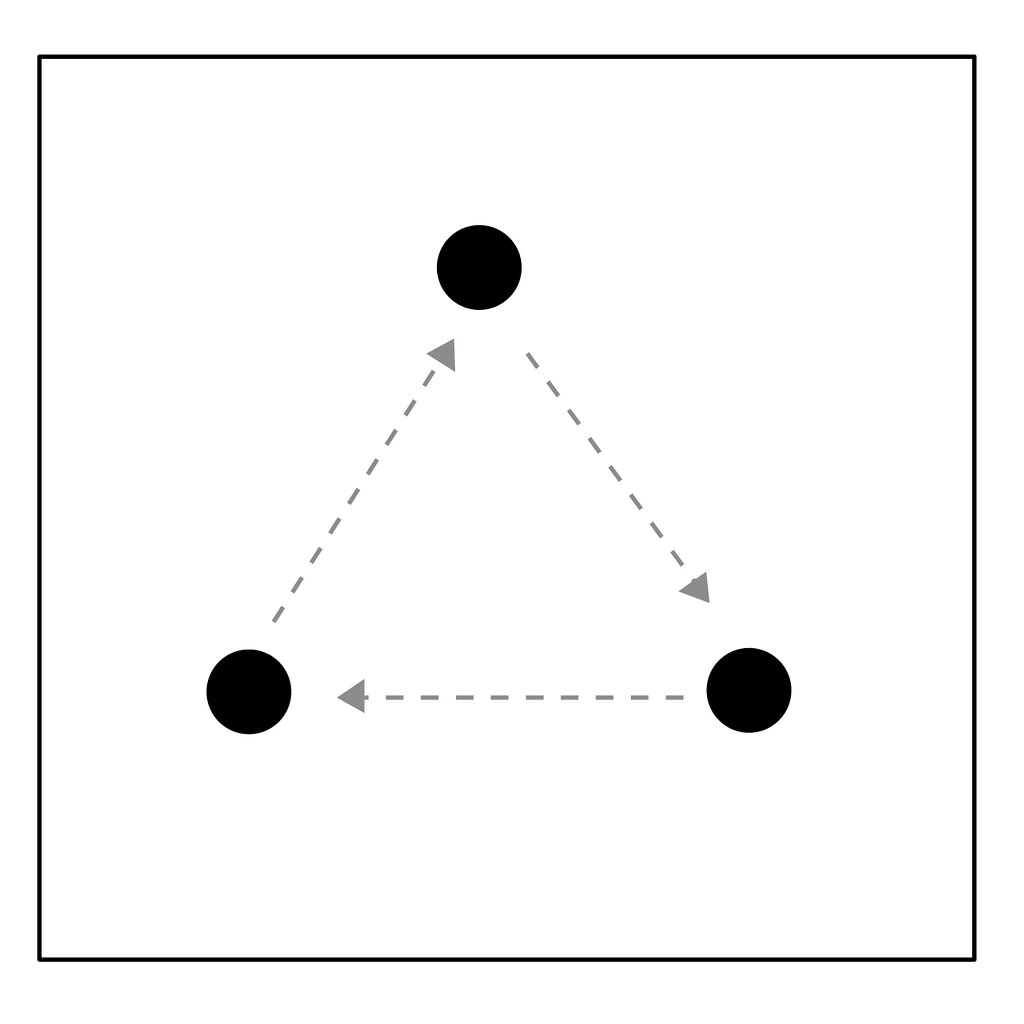The illustration is a meticulously structured square, defined by a thin black line framing its perimeter. Within this frame, three black circles are arranged in a triangular formation, with one circle positioned at the top and the other two at the bottom corners. Connecting these circles, delicate gray dotted lines intersect the space, each culminating in a triangle pointing towards a circle—creating a sense of directed movement.

Starting from the top, the first dotted line extends diagonally downward, ending in a triangle pointing at the bottom right circle. Similarly, another dotted line descends diagonally from the top, directing attention to the bottom left circle with its arrowhead. A final dotted line spans horizontally between the two bottom circles, each end capped with a triangle that points towards the opposite circle.

The circles, lines, and arrows are thoughtfully centralized within the square, leaving ample white space between the black elements and the illustration's edges. This spatial arrangement ensures the components are well-balanced and distinctly noticeable, composed precisely at the core of the image for a clean and focused visual presentation.